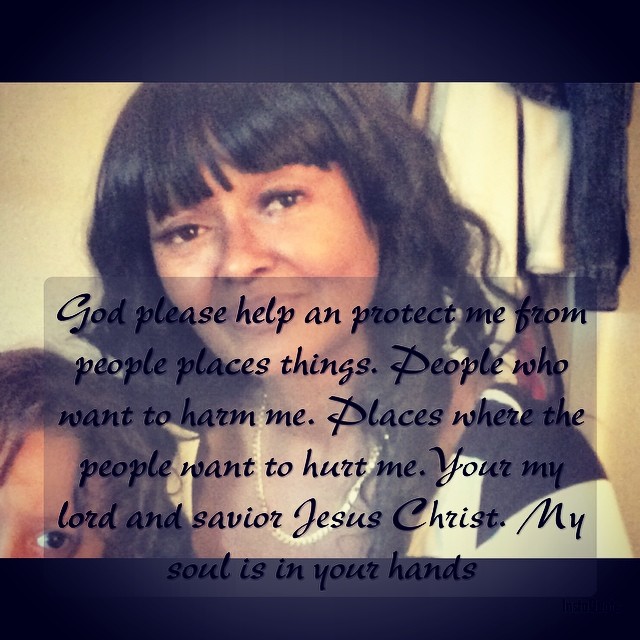This photograph captures a woman with dark hair and short bangs hanging over her face, with a dark complexion suggesting Hispanic descent. She is staring intently at the camera, exuding a sense of urgency and vulnerability. Partly visible beside her is another person whose eye and forehead appear partially in the frame on the right-hand side of the image.

The photograph features a monochromatic color scheme dominated by tan, black, and white tones. The woman is dressed in a black and white shirt and wears a chain, possibly silver, around her neck. Behind her, walls painted yellow provide a muted backdrop, and a black denim-like coat hangs on the wall. There is also a white item hanging that is somewhat out of focus.

Across the image, there are thick black strips at the top and bottom, possibly adding to the sense of confinement or urgency. The bottom of the photograph contains text in black on a gray background which reads: "God please help and protect me from people, places, things. People who want to harm me. Places where the people want to hurt me. You're my Lord and Savior, Jesus Christ. My soul is in your hands." This message underlines the woman's expression of seeking protection and faith, adding a poignant layer to the scene.